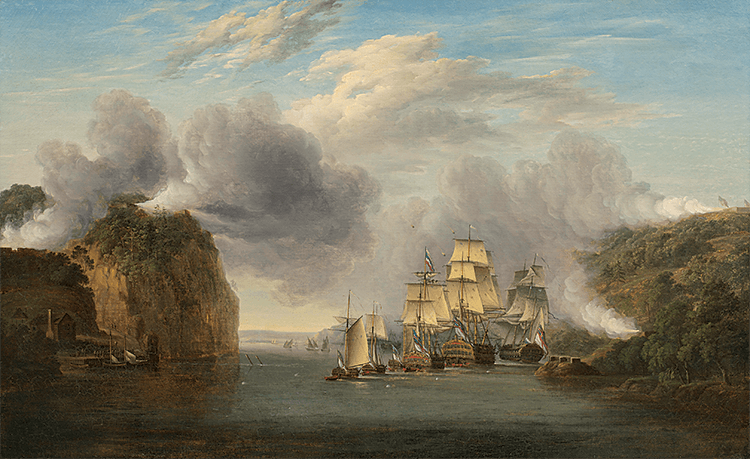The painting depicts a serene yet dramatic maritime scene, likely an oil painting, capturing the essence of a cloudy afternoon at sea. The sky above features a mix of dark gray clouds and white, fluffy clouds, with patches of blue peeking through, hinting at the afternoon sun. To the left, a towering, rocky boulder rises from the water, crowned with sparse greenery, mirrored by a slightly smaller, equally vegetated boulder on the right. 

Dominating the midground, a flotilla of at least six sailing ships, characterized by their raised ivory sails and brown hulls, traverse the calm, gray waters of a canal-like passage. One ship, second from the left, proudly flies the French flag atop its mast. The ships' historical design, with multiple sails and masts, suggests an era from 100 to 200 years ago. In the background, several more ships can be seen, though their details are faint, adding depth to the scene.

On the right side of the composition, a cannon emits a plume of smoke, firing toward the ships, adding an element of action to the tranquil seascape. On the left, a small dock nestles beside the rocky outcrop, with two boats—tinged with bluish-yellow—sailing away into the distance. This rich and detailed imagery captivates, blending natural beauty with human endeavor on the high seas.